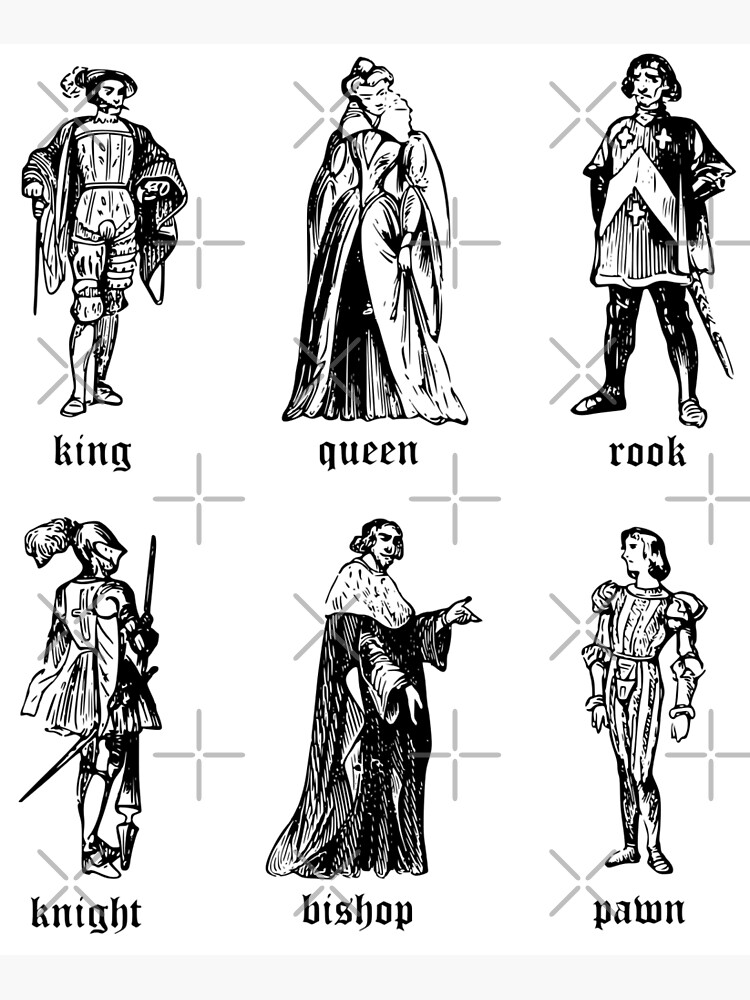This detailed black and white sketch artistically represents chess pieces in human form. The first piece is the King, who is depicted wearing regal armor and a long, flowing robe draped over his shoulders. Adjacent to him stands the Queen, adorned in a floor-length dress with her hair elegantly styled in a bun-ponytail. Following her is the Rook, characterized by a long overcoat that extends just above the knees. The Knight is next in line, fittingly portrayed in attire that suggests readiness for battle. The Bishop is rendered with accouterments that befit a religious figure of authority. Lastly, the Pawns are depicted as simpler, more uniformly dressed figures, embodying their role as the foot soldiers of the chessboard. This intricate and imaginative sketch brings a unique humanized perspective to the traditional chess pieces.